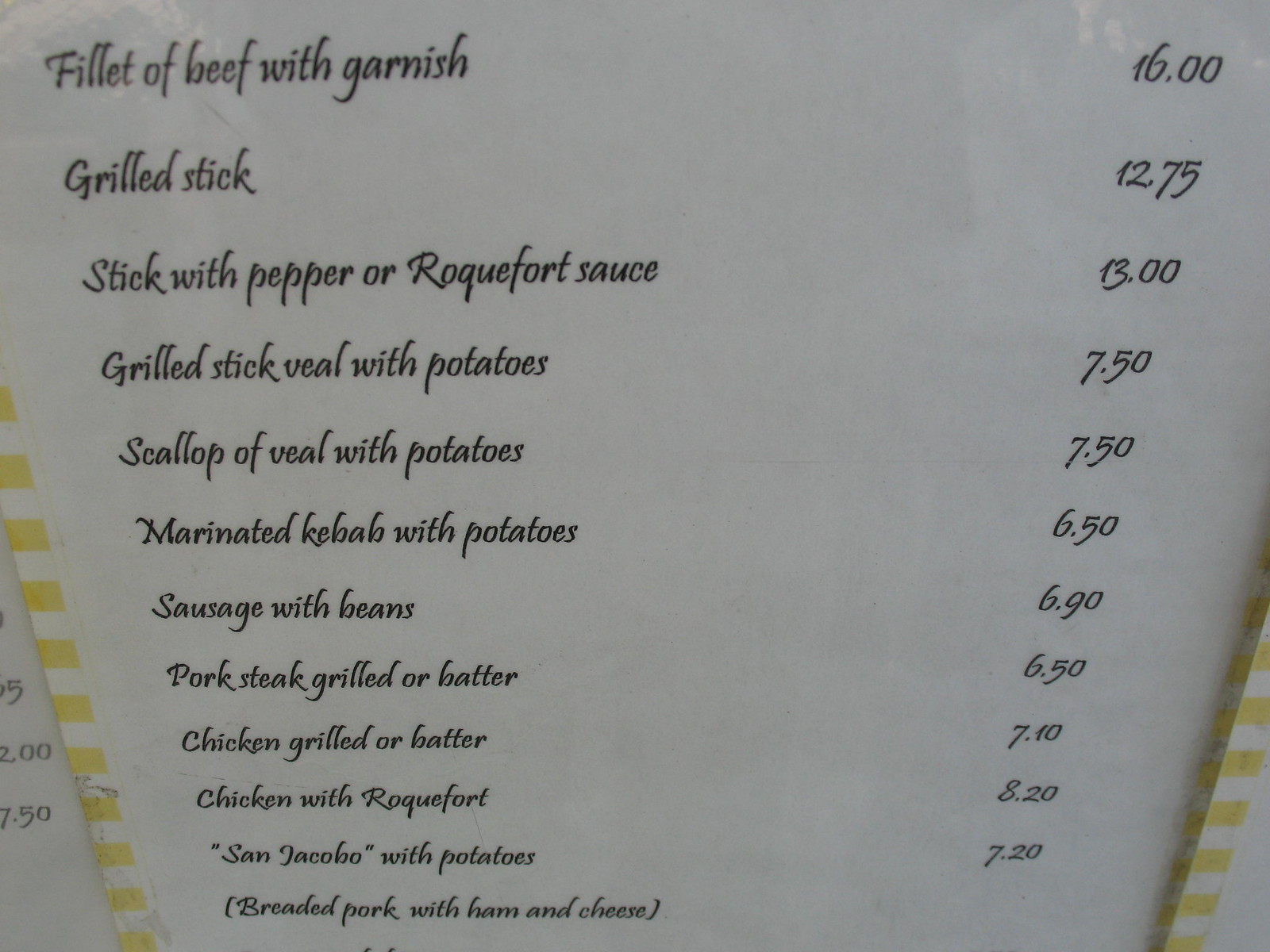The photograph features a menu with a white background and a yellow and white checkered border running along the edges. The black text details a variety of entrees and their prices: Fillet of beef with garnish for $16, grilled steak for $12.75, stick with pepper or Roquefort sauce for $13, grilled stick veal with potatoes for $7.50, scallop of veal with potatoes for $7.50, marinated kebab with potatoes for $6.50, sausage with beans for $6.90, pork steak grilled or in batter for $6.50, chicken grilled or in batter for $7.10, chicken with Roquefort for $8.20, and San Jacobo with potatoes for $7.20. At the bottom, partially cut off, details about breaded pork with ham and cheese can be seen in parentheses. The image is zoomed in, providing a close-up view of the menu categories and their respective prices.